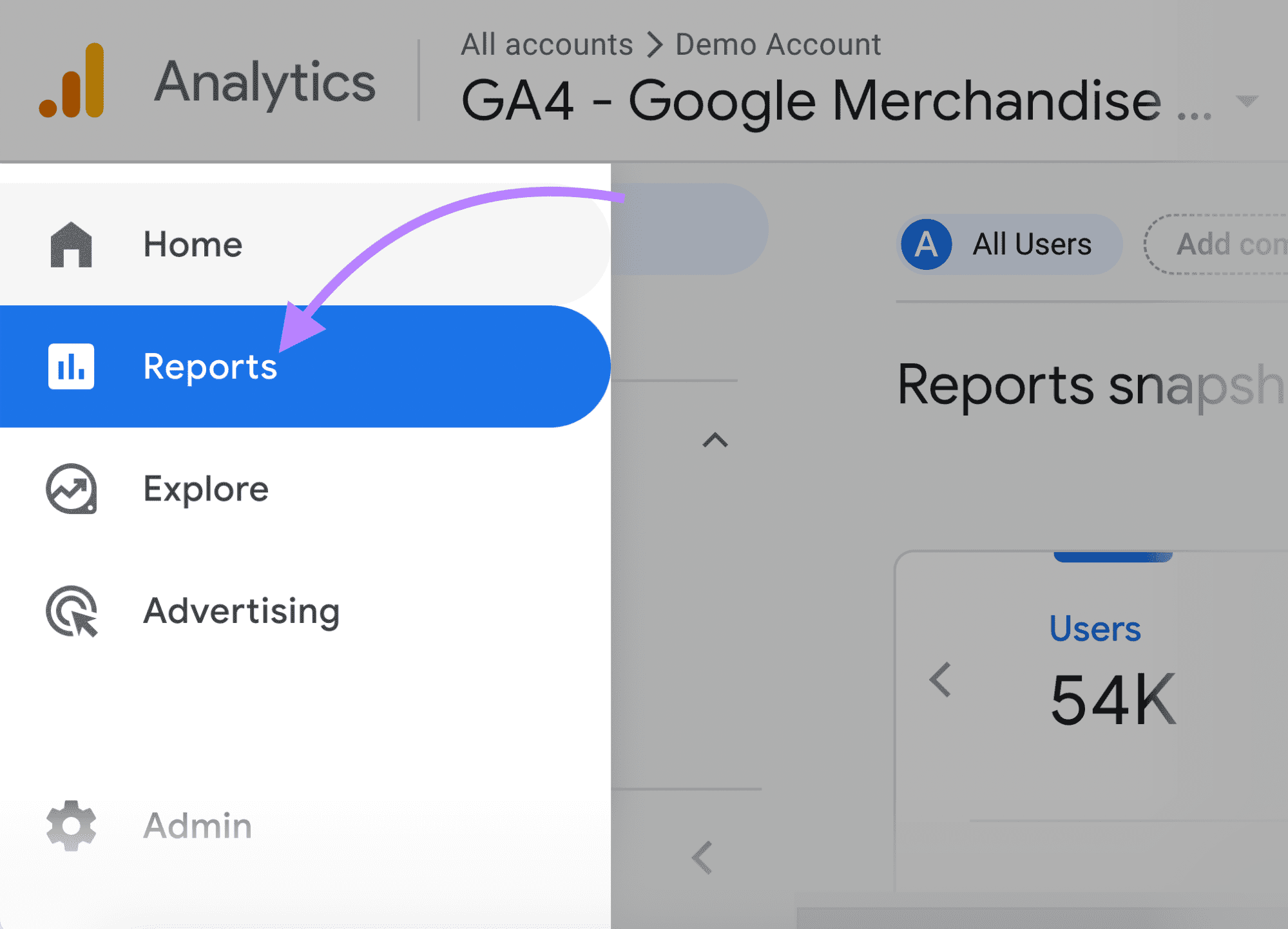This image is a partial screenshot of a Google Analytics interface. The main focal point is a highlighted vertical rectangle on the left side, slightly taller than it is wide. At the very top of this rectangle, there is a section labeled "Home." Below "Home," in white text against a blue background, the word "Reports" is prominently displayed. This section is styled with rounded corners on the right edge. Further down the list, in gray text on a white background, the labels "Explore," "Advertising," and "Admin" are visible.

The remainder of the screenshot is partially grayed out due to the highlighted menu. On the far left, the Google Analytics logo is visible, consisting of three vertical bars—one tall yellow bar, one medium red bar, and a small red dot. To the right of the logo, there is text in capital letters: "GA Dash Google Merchandise."

On the right side of the image, a small portion of the Dashboard is visible. Specifically, in the bottom right corner, there is a blue label that reads "Users," accompanied by a black text indicating "54K."

Overall, this screenshot captures key navigational elements of the Google Analytics interface, highlighting menu options and partially revealing user analytics data.